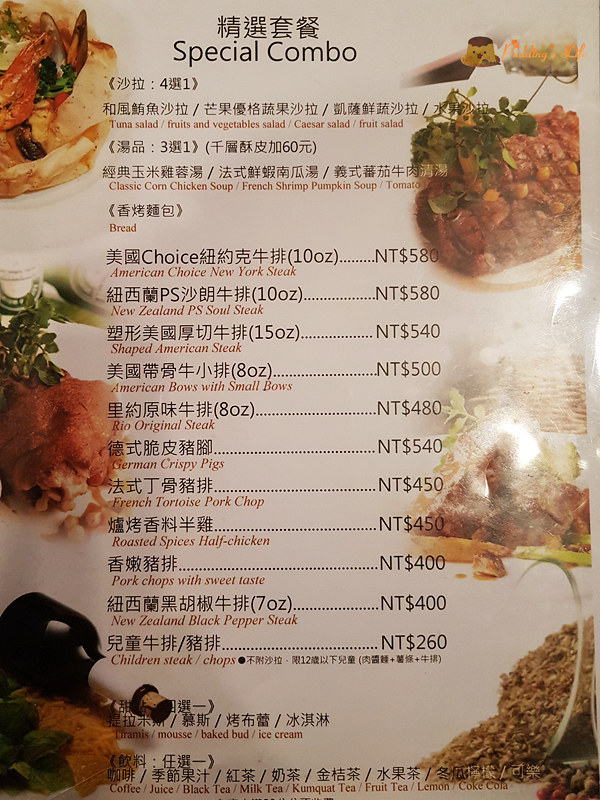This photograph captures a comprehensive menu from an Asian restaurant, prominently featuring a "Special Combo" section. Adorned with Asian characters at the top, the menu's layout transitions beneath into English, listing the appetizing offerings. Surrounding the menu, vibrant graphics of the food items advertised create a visually engaging experience.

On the left side:
- A detailed image of a dish with shrimp
- Below it, a succulent chicken dish
- Further down, a bottle of wine with a cork and a white seal around its neck
- An enticing bowl of rice is depicted near the bottom

On the right side:
- A grilled chicken dish showcasing crisscross grill marks
- An unclear graphic below the chicken dish
- At the bottom, a jar of seasoning spilling out, adding a colorful touch

The menu is set against a pristine white background, ensuring the items and graphics stand out clearly and invitingly.